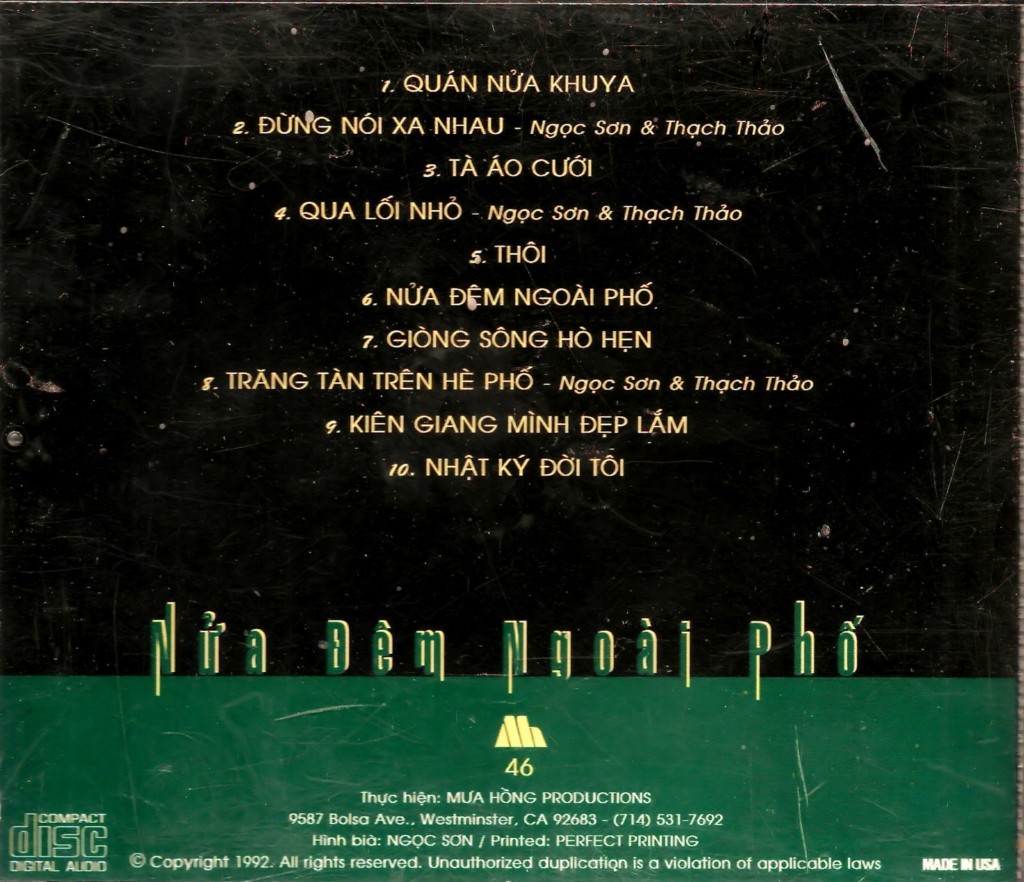The image depicts the back cover of a compact disc (CD) with a list of songs, primarily written in Vietnamese. The design is divided into two main sections: the top 80% features a black background with yellow text, while the bottom 20% has a green background with white text. The CD, identified by the "Compact Disc Digital Audio" label in the bottom left-hand corner, includes a total of 10 songs listed in numerical order, though the specific titles cannot be discerned due to the language barrier. Additionally, the cover provides a copyright date of 1992 and includes an address, "9587 Balsa Avenue, Westminster, California," along with a phone number. The production company is partially identified as "Mookong Productions," and the CD appears to have been made in the USA.